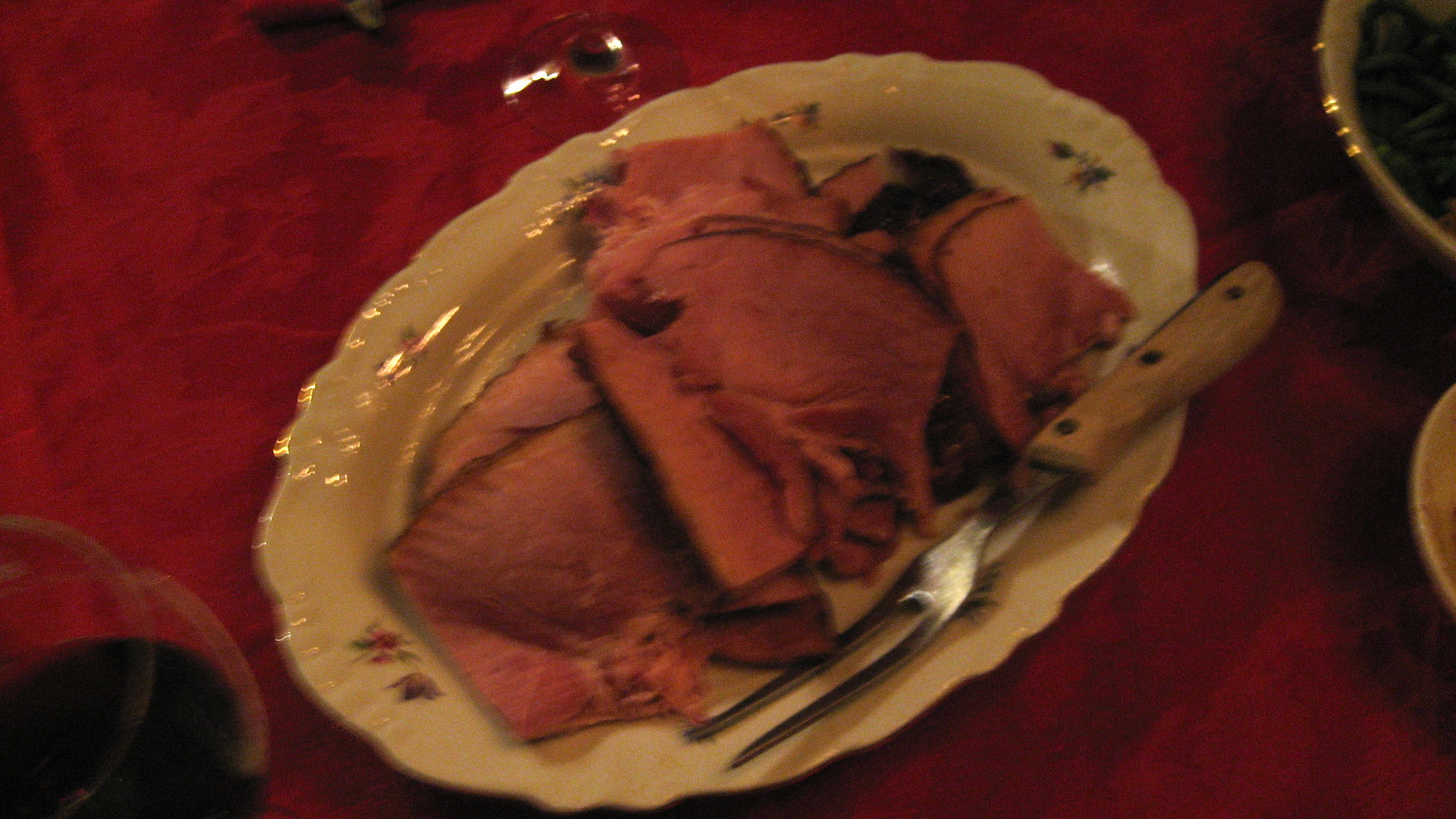The image is a top-down view of an elegantly set meal on a rich, rose-red tablecloth adorned with an intricate floral design. At the center sits an oval, porcelain platter with a delicate floral pattern and gold artwork along the rim. The platter is filled with thinly sliced, well-done roast beef, stacked atop each other, and displaying a crusty edge but no visible fat. Accompanying the meat is a long, two-pronged silver meat fork with a light brown wooden handle. To the left, there is a wine glass filled with a dark red wine, and although the stem is not visible, the cup of the glass is evident. On the right side of the image, partially visible, are two ceramic sauce bowls. One bowl appears green with a gold-tinged edge, and the other is brown with a white interior. This meticulously arranged setting is further complemented by the red tablecloth, creating an inviting and luxurious dining atmosphere.